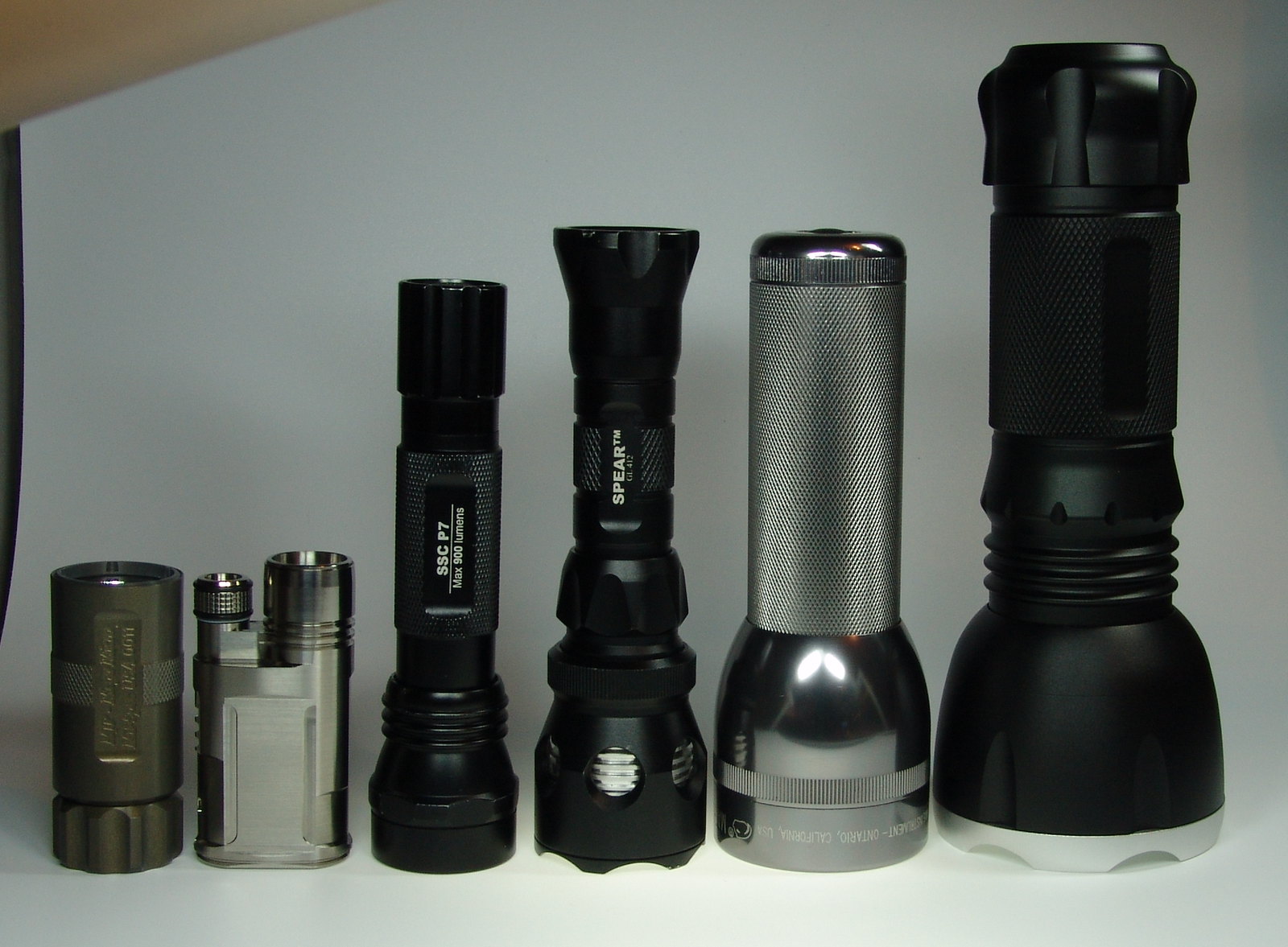The color photograph features a line of six different flashlights arranged from left to right on a white surface. These flashlights vary in size, shape, design, and color. On the far left, there is the smallest flashlight, followed by a slightly larger one next to it. As we move to the right, the flashlights increase incrementally in size: the third and fourth are larger than the previous ones, though the fifth flashlight is slightly shorter, and the sixth one is the largest. The torches are positioned with their lamps facing downwards. The flashlights include three black models, two silver ones, and one in a military dark green color. Some of them feature text such as "Spear" and "SSCP-7." The surface they are placed on appears white, with a slight diagonal line indicating the surface's end at the top left, revealing a blurred, beach-colored background. There is a slight reflection indicating the use of a camera flash.